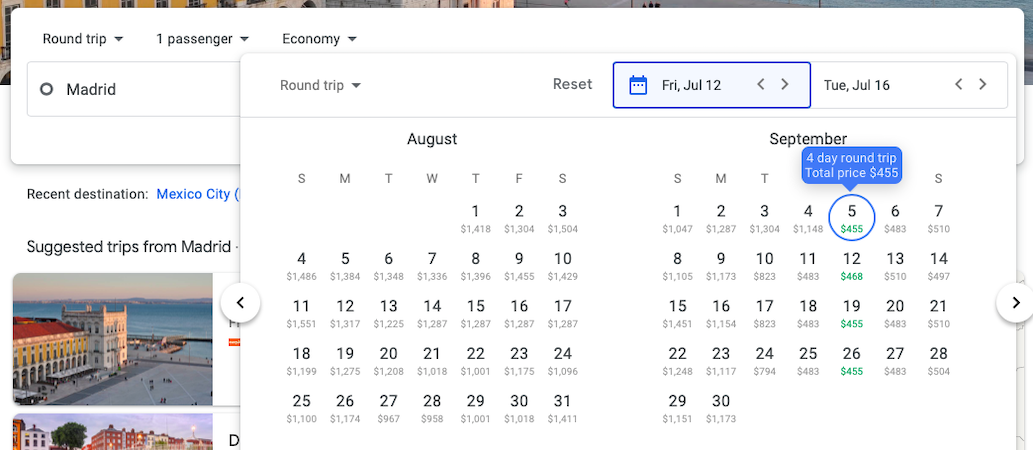**Detailed Caption:**

The image displays an airline ticket booking interface focusing on a roundtrip flight for one passenger in economy class, departing from Madrid to Mexico City. The roundtrip itinerary shows specific travel dates: departing on Friday, July 12th, and returning on Tuesday, July 16th. The interface features a monthly calendar view for August and September, which includes days marked with different colors to indicate varying price levels. A notable element is a blue circle highlighting the number 5. Some dates are marked in green to indicate lower costs. The total price for the four-day roundtrip is listed as $155. The background of the interface is lightly illuminated, offering minimal distraction from the information. The interface seems to be part of an airline's booking system.